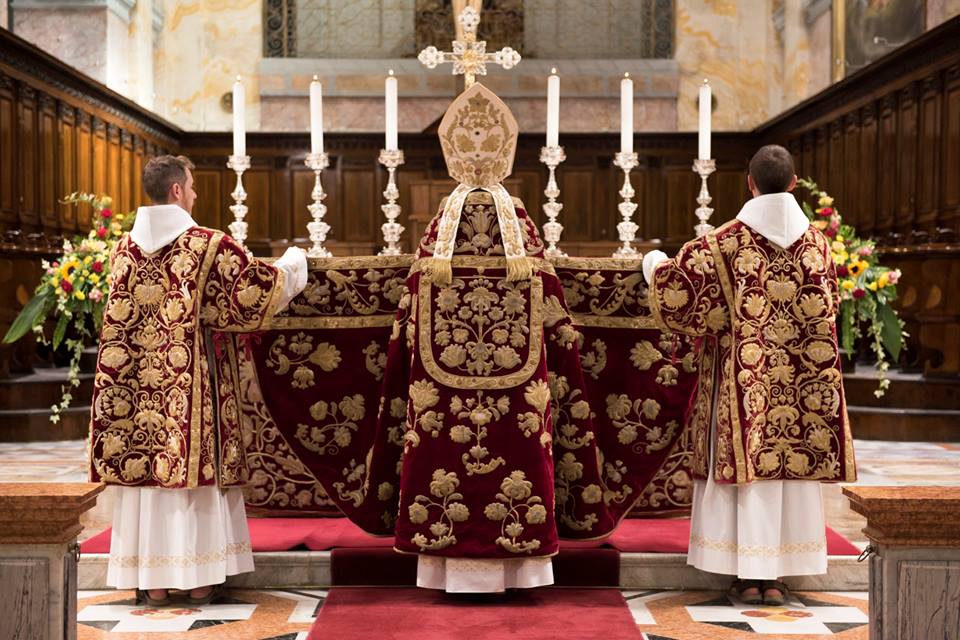In this photograph, taken from the perspective of the congregation inside a cathedral or church, three religious officials, possibly priests, are standing at the altar facing away from the camera. The central figure, distinguished by a large, ornate miter hat, stands between two other priests with short, trimmed brown hair. All three are dressed in richly adorned robes with a burgundy background and elaborate gold embroidery over simple white albs. The two outer priests are seen holding the central priest's ornate robe.

They are positioned in front of an altar, itself draped with a sumptuous red and gold embroidered cloth. The altar features six tall glass candlesticks, each holding a lit white candle, and an ornately embellished gold cross in the center. The setting includes a marble and wooden inlaid backdrop with two pyramidal flower arrangements bursting with yellow and red flowers on either side of the altar.

Below the altar, a red runner carpet creates a T-shape, extending both in front of the altar and down the start of the church aisle, adding to the visual symmetry and sacred atmosphere of the scene.